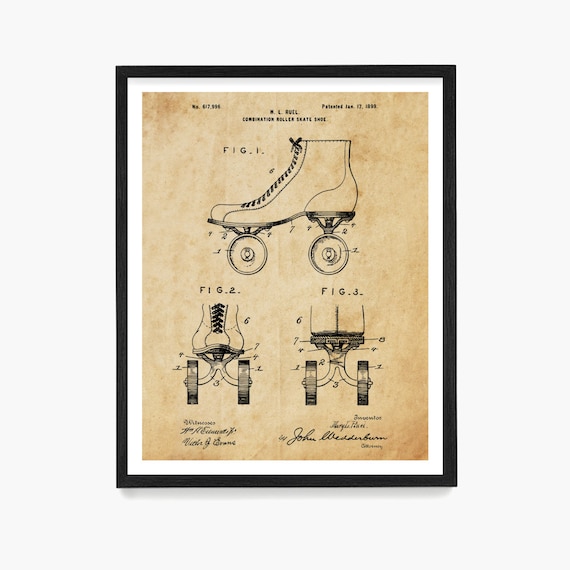The image depicts a vintage, framed diagram of a roller skate, reminiscent of an old patent illustration. The frame is black with a white border, enclosing a piece of yellowish, timeworn paper that adds to the antique aesthetic. The diagram showcases a roller skate from three perspectives: the side (with the toe pointing left and the heel pointing right) labeled as Figure 1, the front labeled as Figure 2, and the back labeled as Figure 3. Each figure is annotated with numbers pointing to various parts of the skate. The illustration is rendered in black and white, capturing the detailed construction of the roller skate, complete with laces and wheels. At the top of the image, there is some text in black font which is partially blurred but seems to include a patent number, "617996," and a date, possibly January 1899. Below this text, there's a label indicating "ML Ruel" or "ML Ruil" and a description, "Combination Roller Skate Shoe." The overall appearance suggests that this piece originates from an old patent office, documenting the invention of this particular roller skate model.